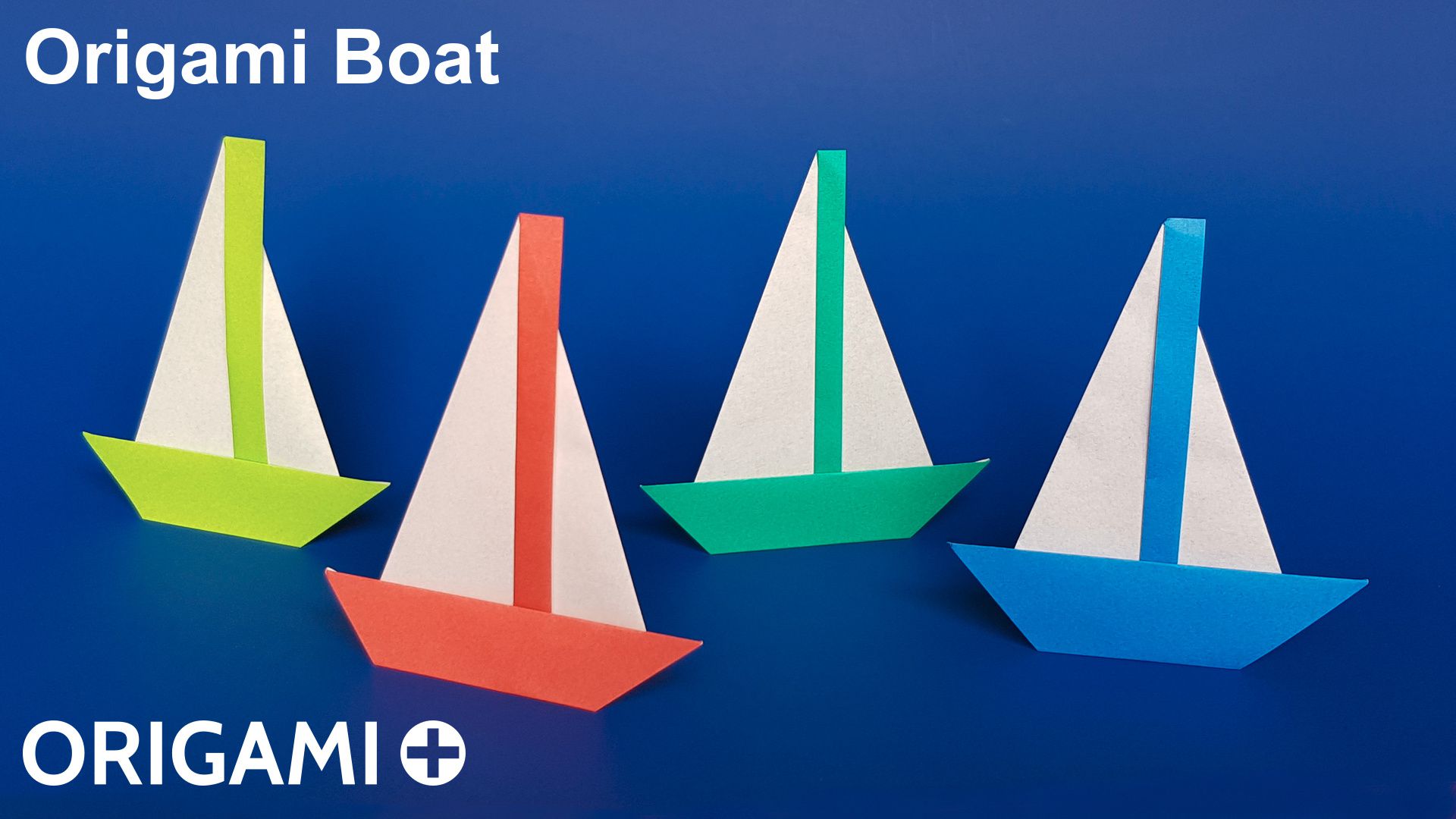The image is a meticulously crafted advertisement for "Origami Plus," showcasing four colorful origami sailboats against a royal blue background. At the top of the rectangular image, the text "Origami Boat" is displayed in a traditional typewriter-style white font, while the bottom features the "Origami Plus" branding with a plus symbol inside a white circle. The sailboats, made from paper, each have white bases with accent colors: lime green, turquoise, red, and blue. They are thoughtfully arranged as if sailing across the page, with the red boat taking the lead, followed by the blue, and the yellow and green boats positioned slightly further back to create a dynamic, freeform layout. The vibrant colors and clear, eye-catching design effectively highlight both the art of origami and the brand, making for an attractive and engaging visual.